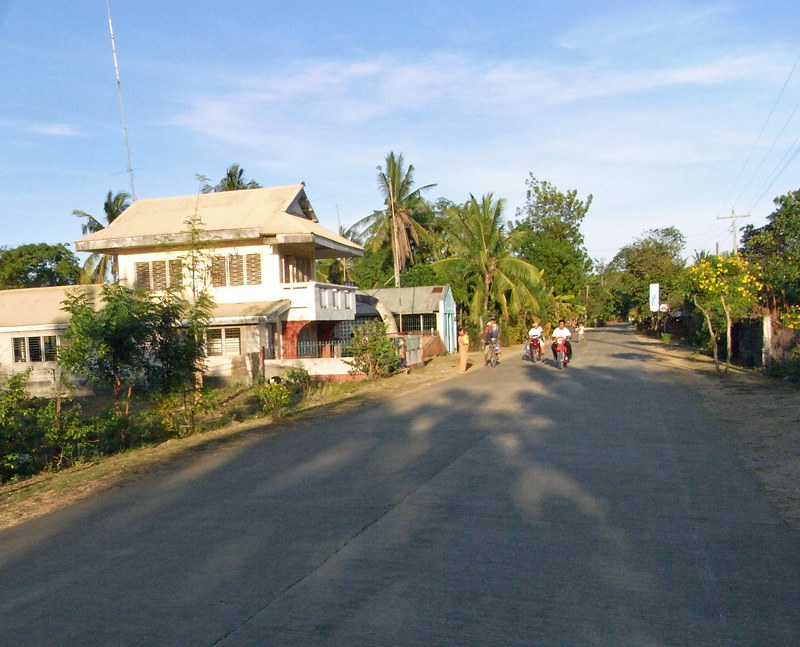The photograph captures a serene residential street, possibly in an Asian or Californian neighborhood, showcasing a large, two-story white house on the left. The house features a reddish rust-colored curve beneath its balcony and a greenish fence enclosing the front yard. A notable garage is also part of the structure. In the background, tall palm trees with generously-sized leaves sway, indicating a coastal or tropical setting. The street is paved and gray, housing minimal signage and power cords, contributing to its clean and uncluttered appearance.

People populate the scene: a woman stands on the edge of the road beside the house, while in the distance, two figures ride bikes and another rides a motorcycle, moving down the street. Additionally, some children are seen playing, enhancing the neighborhood's inviting ambiance. On the right side, a tree adorned with yellow flowers grows near a wooden telephone pole, while a grassy area with some dirt lies beside the road. A white sign can also be spotted in the background.

Overhead wires and a large antenna are visible against the backdrop of late afternoon sunlight, casting long shadows across the scene. The sky is partly cloudy, adding depth to this picturesque and detailed portrayal of a charming residential street.